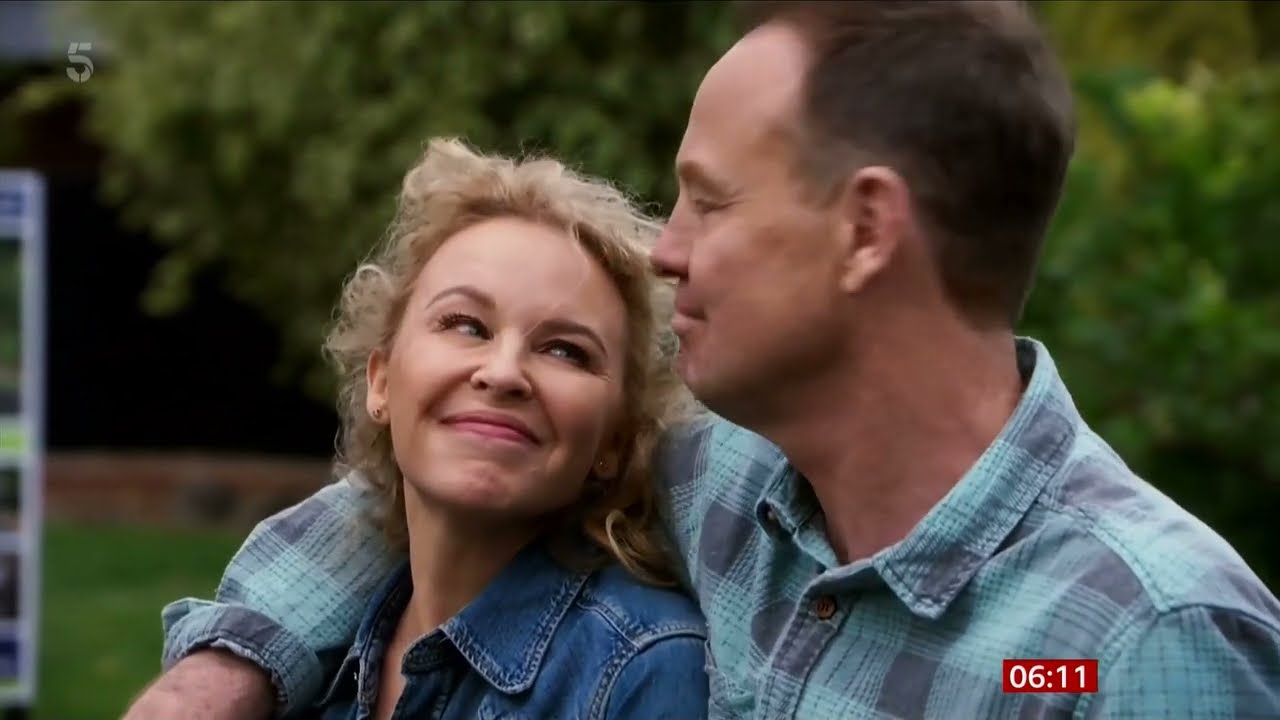In a warmly intimate scene, a man and a woman, both appearing to be in their late 40s or early 50s of Caucasian descent, are captured gazing into each other's eyes with affectionate smiles. The woman, who has short, curly blonde hair, light blue eyes, and pink lips, is clad in a denim collared button-down shirt. She looks up at the man with a quirky smile, while he, with short brown hair, exhibits a closed-mouth smile that creates charming crow's feet around his eyes. The man, wearing a turquoise and gray plaid long-sleeve shirt with a collar, has his right arm affectionately draped over the lady's shoulders. The background showcases a blurred, outdoor scene with trees and grass, drawing focus to the couple. In the lower right corner of the image, a red rectangle with white text displays "06:11," adding a timestamp-like detail to this captured moment of connection.